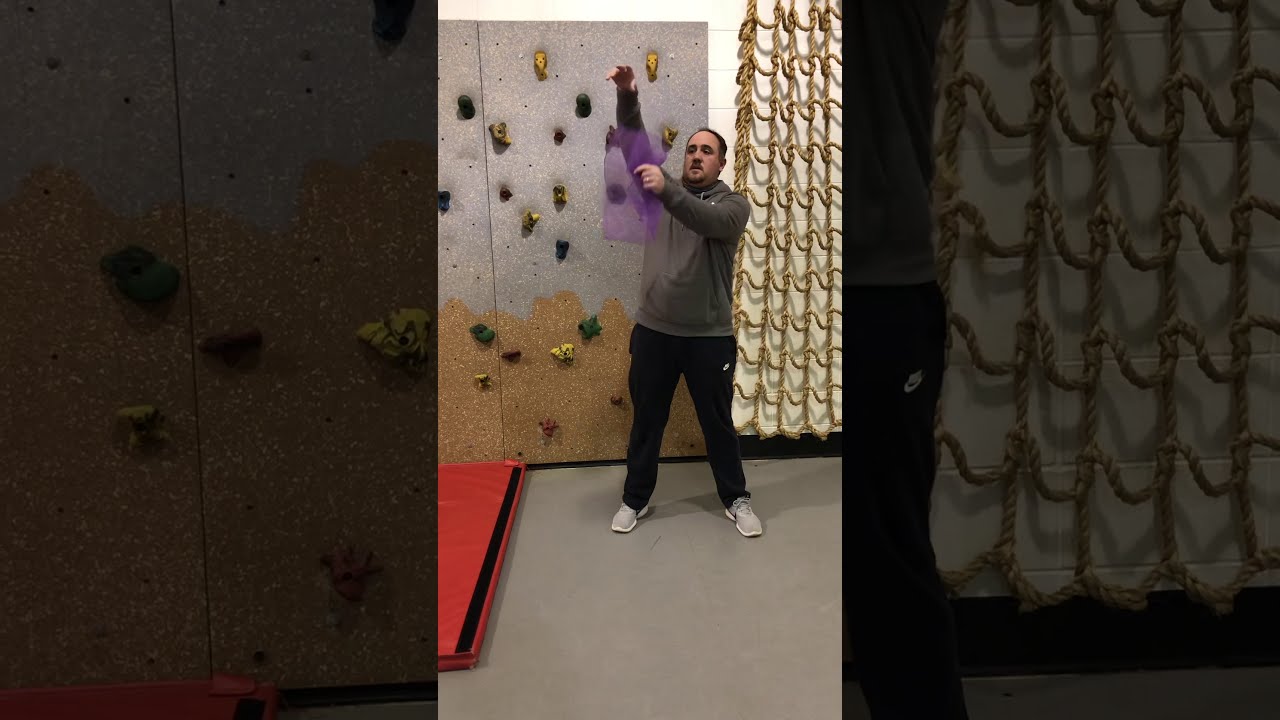This is a detailed photograph of a man in his 30s, standing indoors, presumably in a climbing studio. He is wearing a long-sleeve gray sweatshirt, black pants, and gray shoes. The man has a short-cropped, balding dark hair, and sports a brown mustache and goatee. His right arm is raised, while his left hand holds a translucent purple fabric or plastic square. 

The setting features a climbing wall behind him, adorned with colorful climbing holds in yellow, green, red, and blue. To the right of him, there is a series of tan ropes arranged for vertical climbing. The climbing wall has a gray and brown base, and the floor beneath is gray with a red safety mat visible in the bottom left corner of the image, which also has a piece of black Velcro on it. 

Further enhancing the background, there is also a window with white and gold curtains that suggest a mixture of natural and synthetic lighting in the room. Positioned slightly to the right and centered in the frame, this man appears to be demonstrating or explaining something in a presumably organized setting, possibly a gym or climbing class.